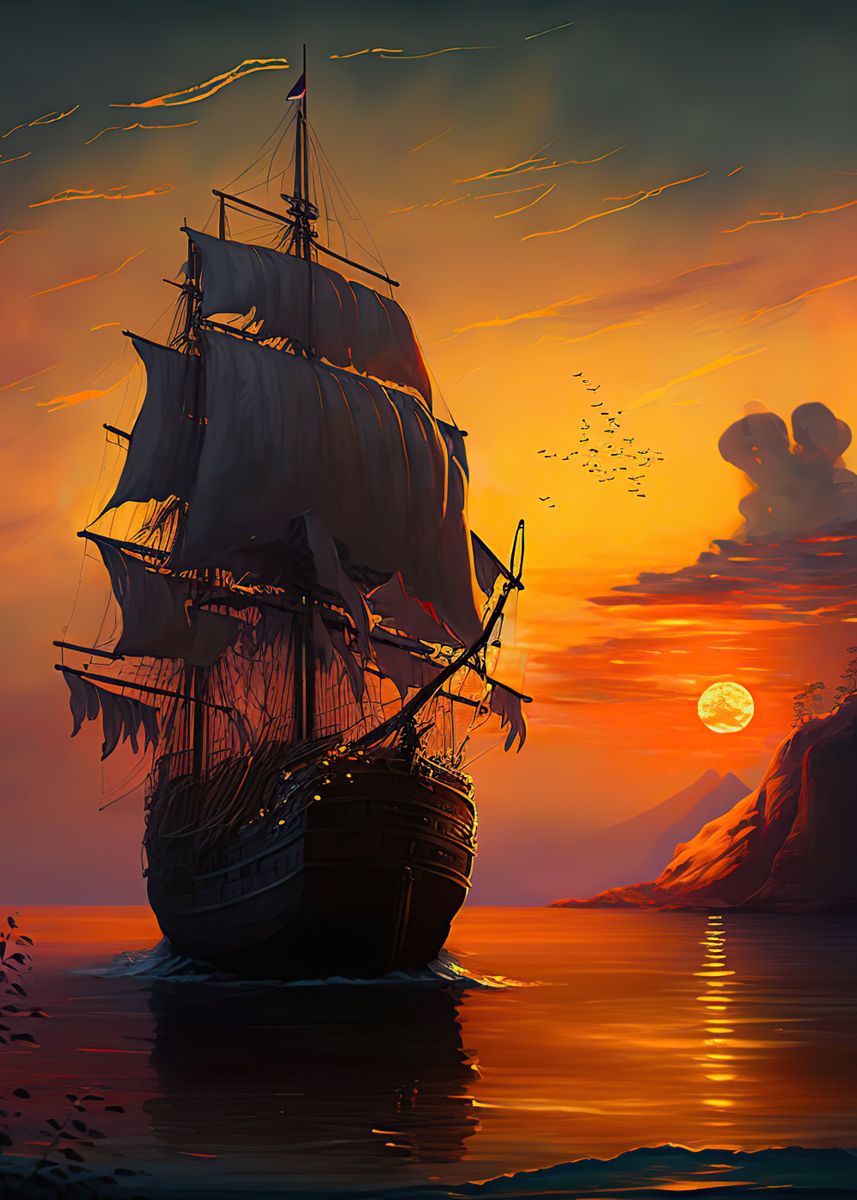The digital artwork portrays a dramatic sunset scene over a calm ocean, bathed in deep hues of orange, red, and yellow transitioning into a dark blue-green sky. The vibrant colors are reflected in both the water and the dark, ominous clouds that loom in the sky. Prominent in the scene is a large, weathered pirate ship positioned to the left, sailing towards the viewer, seemingly pulling into a bay or cove. The ship, dark and silhouetted, features multiple masts adorned with tattered sails, swaying as if caught in a strong breeze, and numerous ropes hanging down. It is an old vessel, with parts of its wooden structure missing and worn. A flock of seagulls flies nearby, adding life to the scene. In the distance, large mountains form the horizon, their outlines faintly visible in shades of dark red and purple. Closer mountains with reflective yellow glows and a small hill towards the right of the image frame the scene, suggesting a blend of nature’s ruggedness with the sea’s vast expanse. Reflections of the fiery orange sun dance on the rippling water, further enhancing the image's moody and evocative atmosphere.